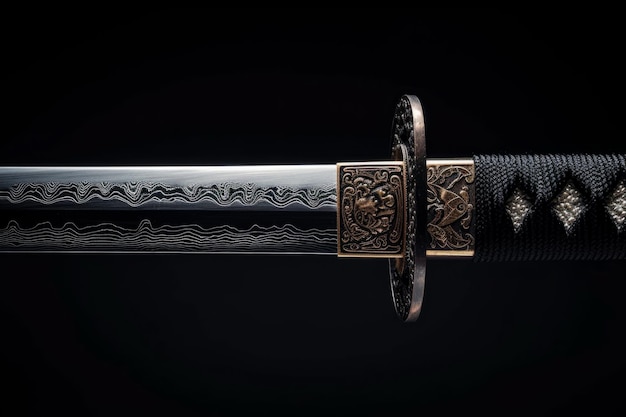The close-up photograph showcases a segment of a traditional Japanese katana against a nearly black background. The focus is on the ornate hilt and hand guard, known as the tsuba, which is a circular, gold-hued metal disc intricately engraved and positioned between the handle and the partially visible blade. The katana's handle is wrapped in black cloth with an intricate, traditional diamond-patterned knot that exposes a textured, white leathery material beneath. The blade itself, a striking silver with a ribbon-like wave pattern indicative of folded steel forging, extends a few inches into the frame, emphasizing the craftsmanship. The overall image captures the artistry and detail of this iconic weapon, with reflections accentuating the blade's polished surface.